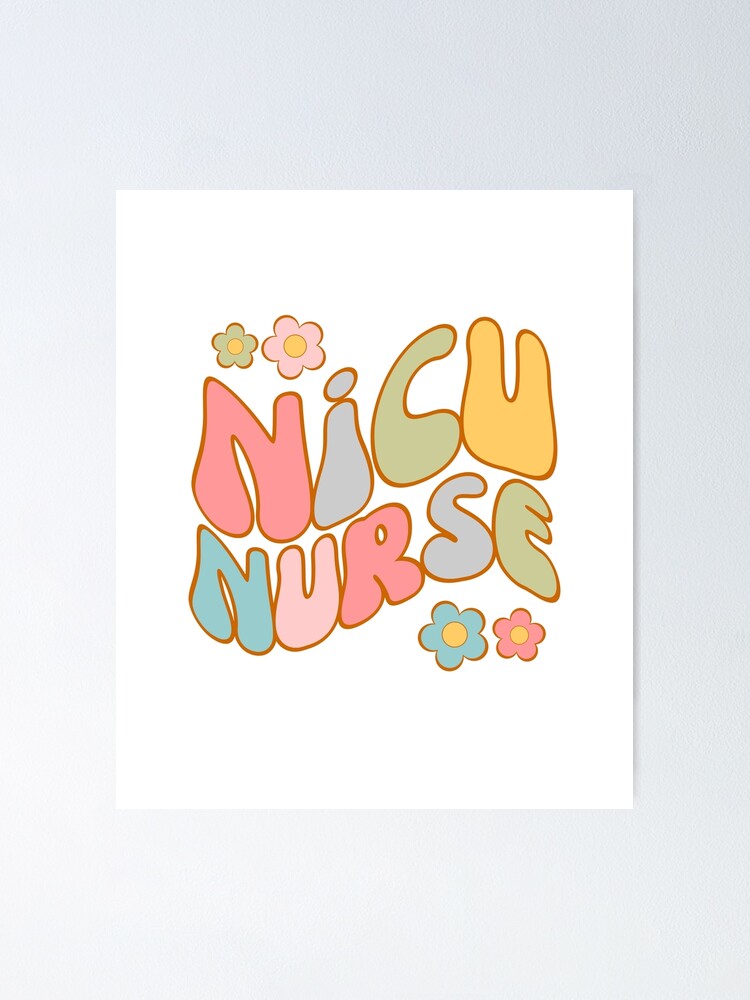The image depicts a white piece of paper lying on a white surface, featuring the large, bulbous text "NICU" across the center, with "Nurse" written directly underneath. The letters in "NICU" are colored sequentially in pink, blue, mossy green, and yellow, while the letters in "Nurse" are colored blue, light pink, red, blue, and a grayish-green. Near these words, there are four flowers; two are positioned above the 'N' in "NICU," with the left flower being green and the right one pink. Below the 'S' and 'E' in "Nurse," there are two more flowers, the left being blue and the right being pink. In addition, the entire scene is set on a rectangular background that has both pale blue and gray hues.